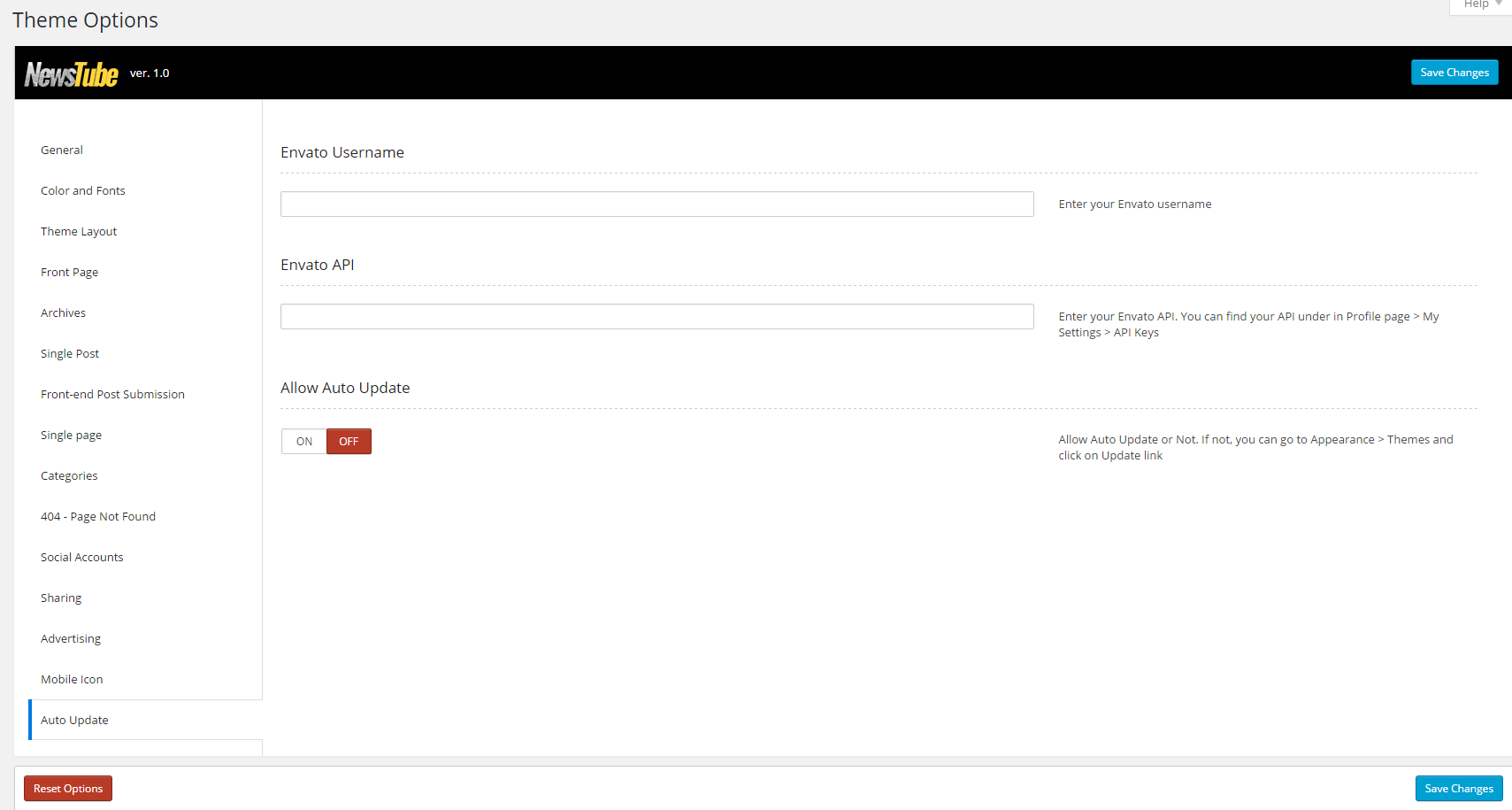The image depicts a settings interface for a web application. At the top, there's a gray border labeled "Theme Options." Below this, a prominent black box displays "News Tube Version 1.0." On the far right side of the black box, a blue button labeled "Save Changes" is visible.

On the left side of the interface, a vertical sidebar menu lists multiple options: General, Color and Fonts, Theme Layout, Front Page, Archives, Single Post, Post Submission, Single Page, Categories, 404 Page Not Found, Social Accounts, Sharing, Advertising, a Mobile Icon, and Auto Update.

To the right of the sidebar menu, there's a section labeled "Envato Username" with a segmented line running horizontally below it. Under this line, a text box prompts users to "Enter your Envato username." This section appears to be dedicated to integrating or validating the user's Envato account details.

The interface is designed with a clean and organized layout, facilitating easy navigation and customization for users managing their news-based web content.